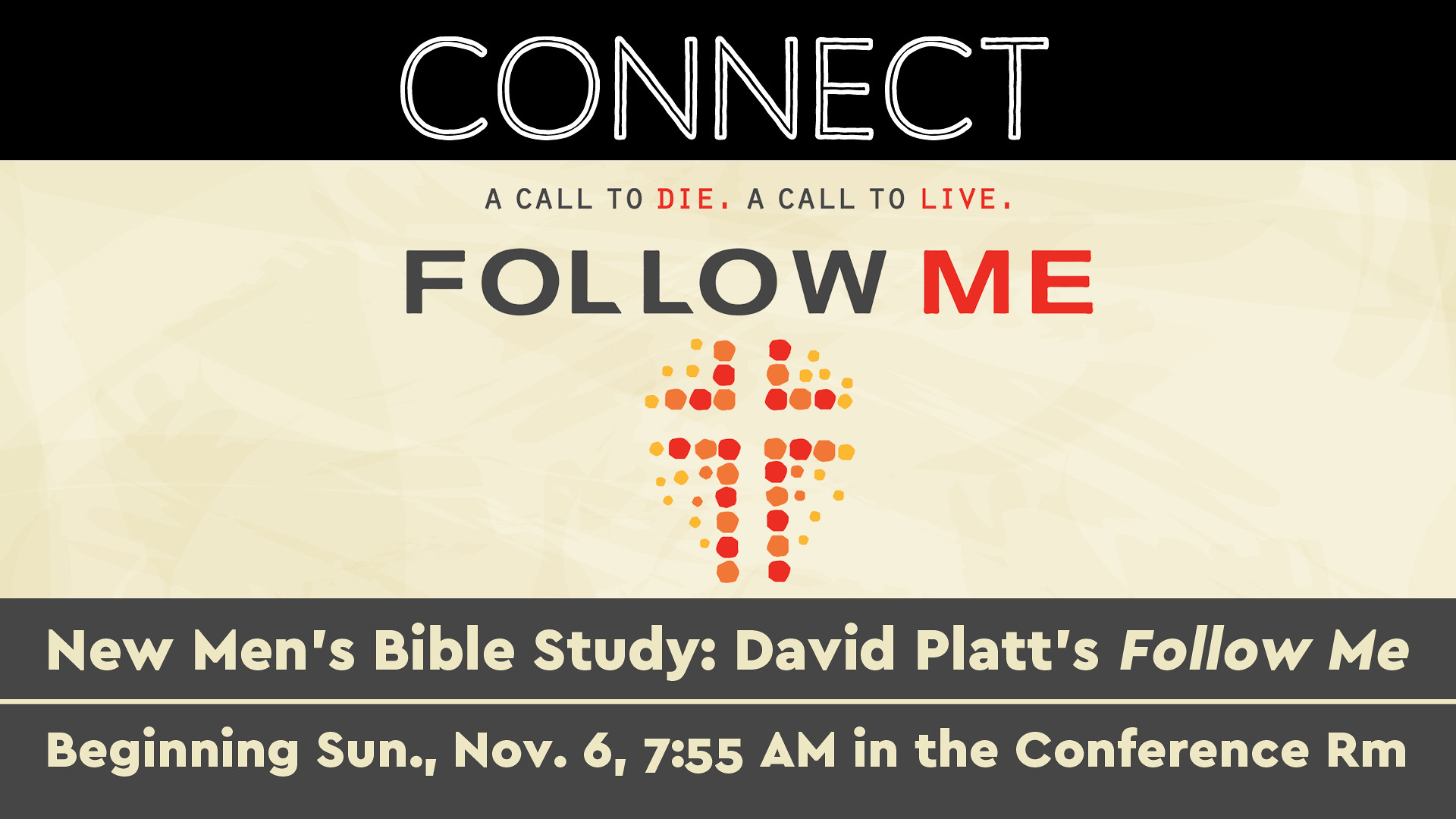The image is a horizontal, color-infographic advertisement for a new men's Bible study group. At the top, there is a black banner with a white text, featuring the word "CONNECT" in all caps with a black line through each letter. Below this, a light brown banner contains the phrases "A CALL TO DIE," "A CALL TO LIVE," and "FOLLOW ME" centered vertically. In these phrases, the words "DIE," "LIVE," and "ME" are highlighted in red, while the rest of the text is in gray. Immediately beneath is an outline of a cross formed by circles in shades of orange, red, and yellow. Further down, two dark gray horizontal banners feature cream-colored text that announces the Bible study details: "NEW MEN'S BIBLE STUDY: DAVID PLATT'S FOLLOW ME" and "BEGINNING SUN NOV 6, 7:55 A.M. IN THE CONFERENCE R.M." The background behind the central text and image resembles cream-colored parchment, tying the design elements together into a coherent visual theme emphasizing connection and commitment.